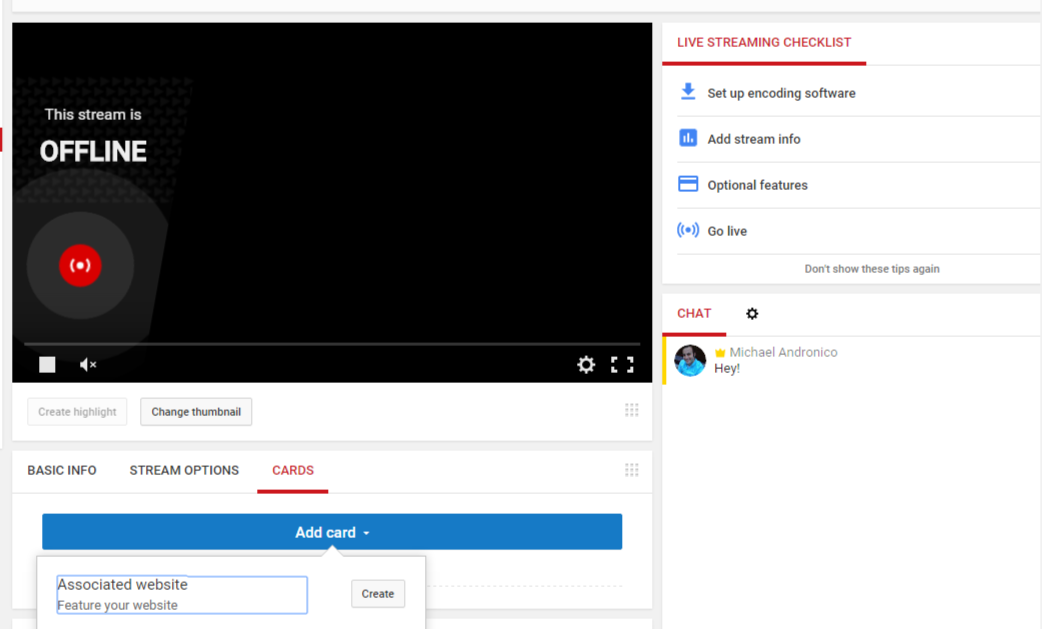A still image from a YouTube live stream interface displays a “Stream Offline” status against a white backdrop. In the upper left corner of the image, a black screen mimics a YouTube player with “This stream is offline” written in white. Below it is an icon featuring a red circle with a white line flanked by a dark gray circle, resembling a recording indicator encircled by a graphical cupcake-like shape.

To the left of the screen, a white box appears next to the volume control button beside another box holding a white gear icon. Next to these controls, another white box states “Create Highlights” in gray, followed by another box declaring “Change Thumbnail” in bold black text.

Beneath these options, black text reads “Basic Info” on the left, “Stream Options” in the center, and “Cards” highlighted in red on the right with an underline. Beneath “Cards,” a long blue bar marked “Add Card” in white text stands out prominently. A pop-up box below this bar contains a white highlighted bar outlined in blue with the words “Feature your website” written in black inside. To its right is another white bar with the label “Create” in black text.

At the top of the page, the red text “Live Streaming Checklist” is flanked by a blue downward-pointing arrow to its right, indicating the setup instructions for encoding software. Below, a blue box with white lines labeled “Add Stream Info” appears to the right of a smaller image of a blue credit card and black text reading “Optional Features.”

Further down, a blue circle icon with two blue lines on either side sits next to the phrase “Go Live” in black. Beneath this, and slightly off-center, the phrase “Don’t show these tips again” is written in black.

Towards the bottom left of the image, a red “Chat” label is accompanied by a black gear icon on its right. Underneath this section is a circular profile picture of a person wearing a blue shirt beside a yellow crown icon. The text “Michael Anthony and Aniko” appears next to the chat icon, along with a comment saying, “Hey!” indicated by an exclamation point.